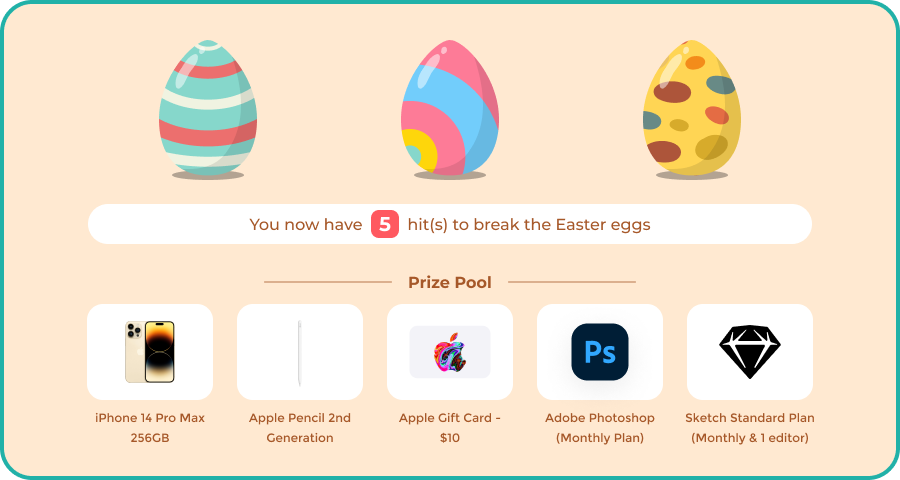**Detailed Description:**

The screenshot displays a minimalistic design featuring a rectangular layout adorned with a thin green line border. Within this rectangle, the background is a soft peach color. At the top, the first row showcases images of three artistically decorated eggs, reminiscent of Easter eggs. 

1. The first egg is intricately striped with a pattern consisting of alternating turquoise, white, coral, and turquoise stripes.
2. The second egg presents a playful color scheme with alternating sections of pink, white, blue, pink, a small segment of yellow on the left, and turquoise.
3. The third egg stands out with its yellow base, covered with a variety of red, blue, gold, and orange spots.

Below these egg images, there is a white banner containing the text: "You now have five hits to break these eggs."

The subsequent section is labeled "Prize Pool" and consists of five distinct squares, each depicting a prize:

1. The first square displays an image of an iPhone with the caption "iPhone 14 Pro Max 256GB".
2. The second square features an Apple Pencil, described as "Apple Pencil 2nd generation".
3. The third square shows an Apple Gift Card labeled "$10 Apple Gift Card".
4. The fourth square includes a smaller square with a black background and blue letters "PS," annotated with "Adobe Photoshop (monthly plan)".
5. The final square contains an image of a black diamond with white highlights, labeled "Sketch Standard Plan, monthly, and one editor".

This detailed caption provides a comprehensive description, shedding light on the simple yet vivid visual elements and the prize offerings within the screenshot.